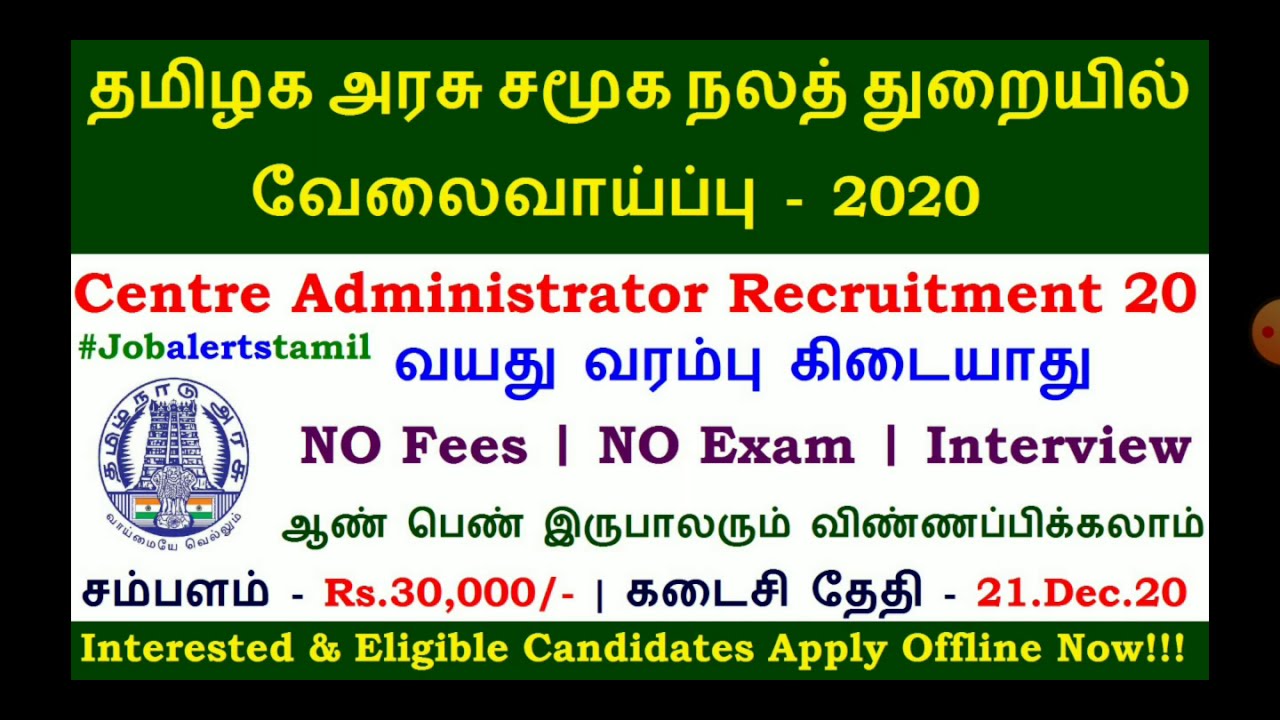The image is of a digital advertisement that resembles a business card, characterized by a prominent green background with text primarily in an Indian language. The entire image is framed by a thick black border. At the top, yellow text is displayed against the green background with curvy lines and dots typical of the script. Beneath this, a white banner features English text in red that reads "Center Administrator Recruitment 20." The line below, in blue text, includes the hashtag "#jobalertstamil," followed by additional text in the Indian script. Further down, the advertisement states in bold letters, "NO FEES, NO EXAM, INTERVIEW." On the left side, it displays "RS. 30,000/-" indicating the salary, and next to it, the date "21.December.20." At the bottom, it urges, "Interested and eligible candidates apply offline now!!!" in enthusiastic punctuation. The image also contains secondary graphics including a tower with symbols, a statue alongside flags in orange, yellow, and green, further adorned with writings underneath.